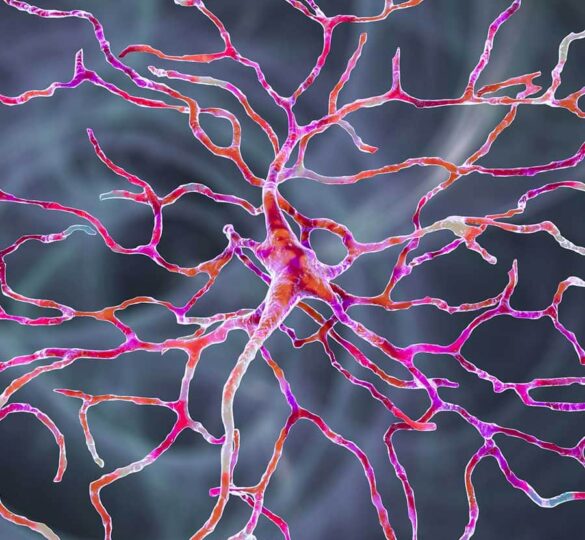This detailed image appears to depict a 3D model or an extreme microscopic close-up of a complex network of blood vessels. At the center of the photograph, a thicker cluster of vessels is prominent, branching out into smaller ones that reach into every corner of the image, filling the entire space. The vessels are varied in color, including shades of red, hot pink, reddish-orange, light purple, and some transparent areas. These colors blend seamlessly together, creating a vibrant and intricate pattern reminiscent of tree roots or lightning strikes. The background is an unfocused, smoky blend of white, gray, and black, with a secondary, blurry network of white veins adding depth to the composition. The image, devoid of any text, people, animals, or man-made structures, possesses an abstract and intriguing quality, making it the type of illustration one might find in a scientific textbook.